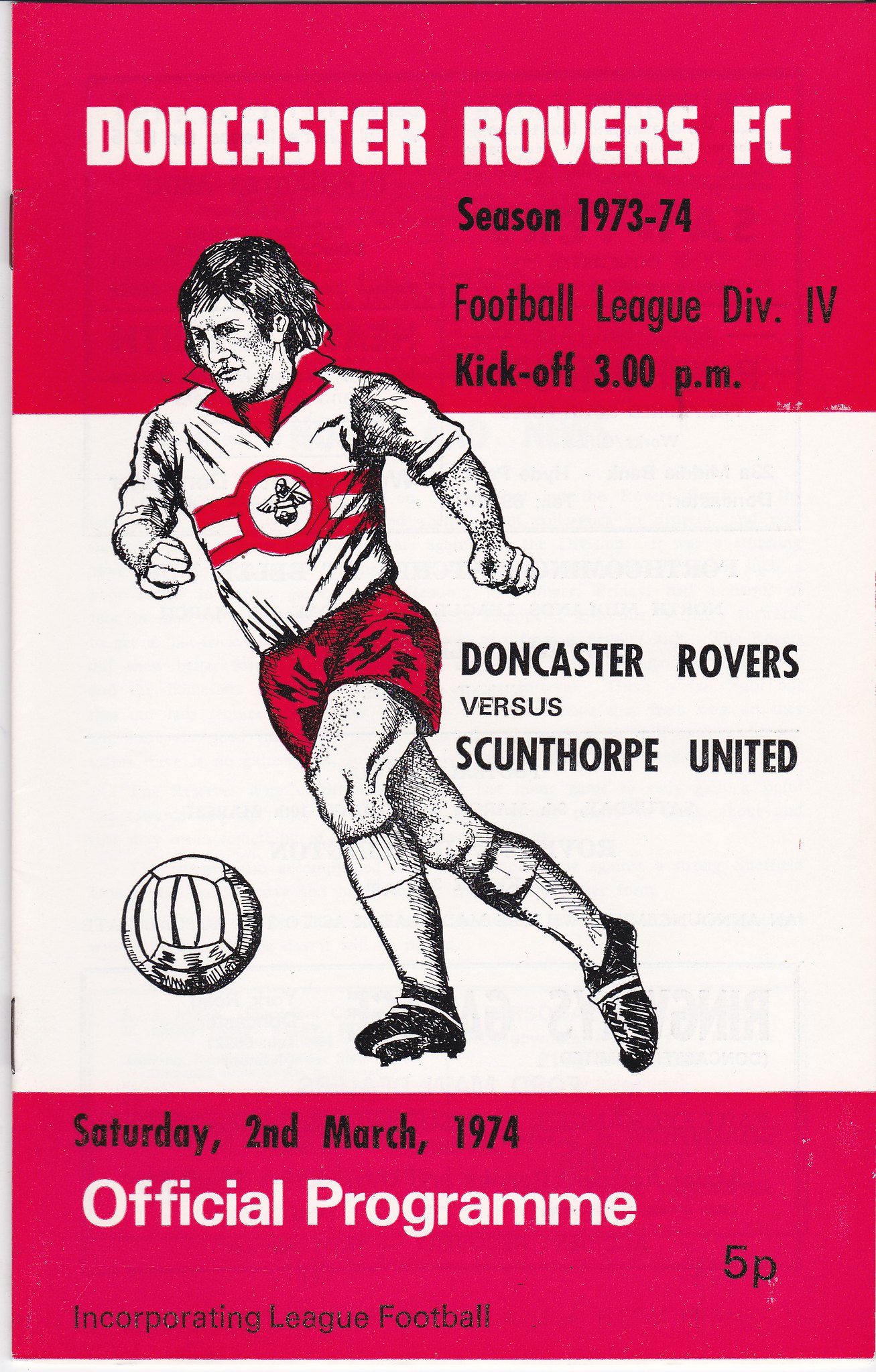The cover of the Doncaster Rovers F.C. official match program for the 1973-74 Football League Division 4 season, dated Saturday, March 2, 1974, features a detailed illustration of a player in action. The athlete, who has dark hair, is depicted wearing a white shirt with a red collar, a couple of red stripes, and the Doncaster Rovers logo in the center, paired with red shorts, white socks, and black shoes. The image, which is taller than it is wide, is divided into a top third header and a bottom fifth footer, both colored in reddish-pink, with a white central background. The top header, in white text with black accents, reads "Doncaster Rovers F.C., Season 1973-74, Football League Division 4, Kickoff 3 p.m." The bottom footer, in black and white text, states "Saturday, 2nd March 1974," "Official Program," "Five Pence," and "Incorporating League Football." The staples binding the program are visible on the left side. To the right of the player, it announces the matchup: "Doncaster Rovers vs. Scunthorpe United."